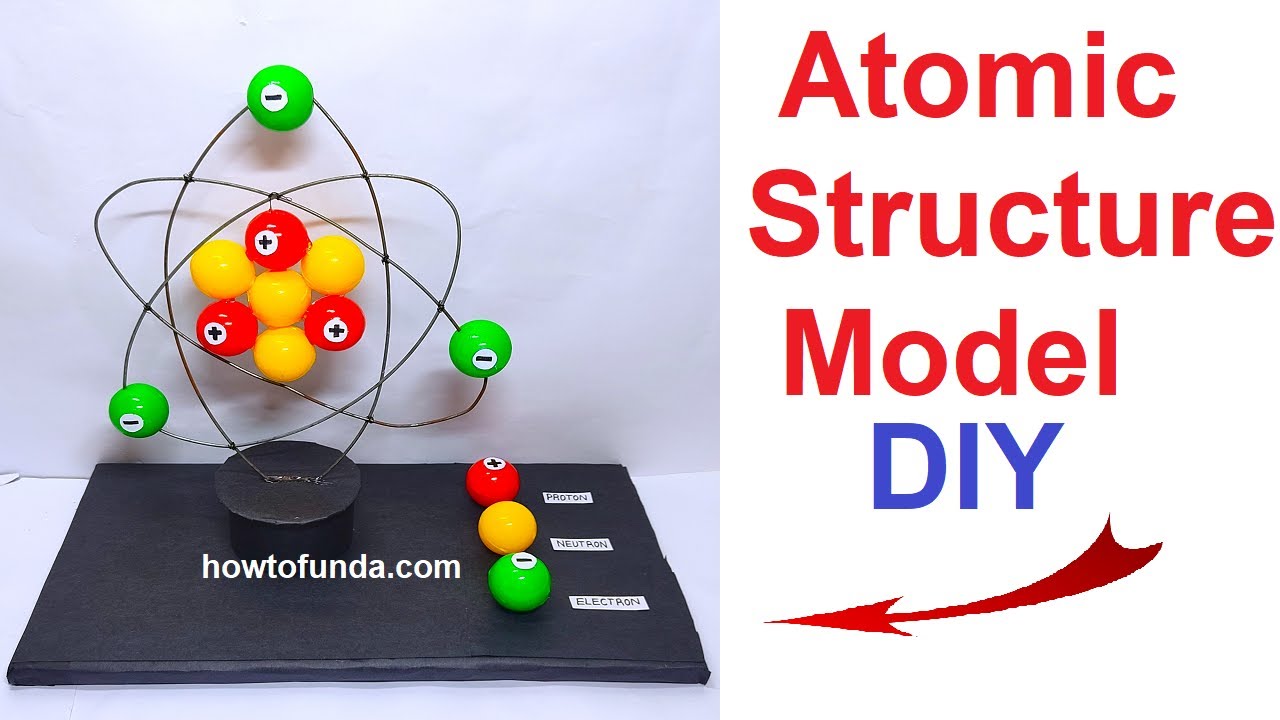The image showcases a detailed, handmade model of an atomic structure, likely created as a school project. The model prominently features text reading "Atomic Structure Model DIY," with "DIY" highlighted in blue, accompanied by an arrow pointing to the left. The components of the atom are color-coded: red balls represent protons, yellow balls represent neutrons, and green balls signify electrons, all orbiting around a central nucleus. These spheres are affixed to metal wires forming the axes, giving the model a structured appearance. Notably, the bottom of the project bears the label "howtofundaid.com." The model appears to be set against a blackboard background, with various labels provided for clarity, making the educational intent of the project clear.